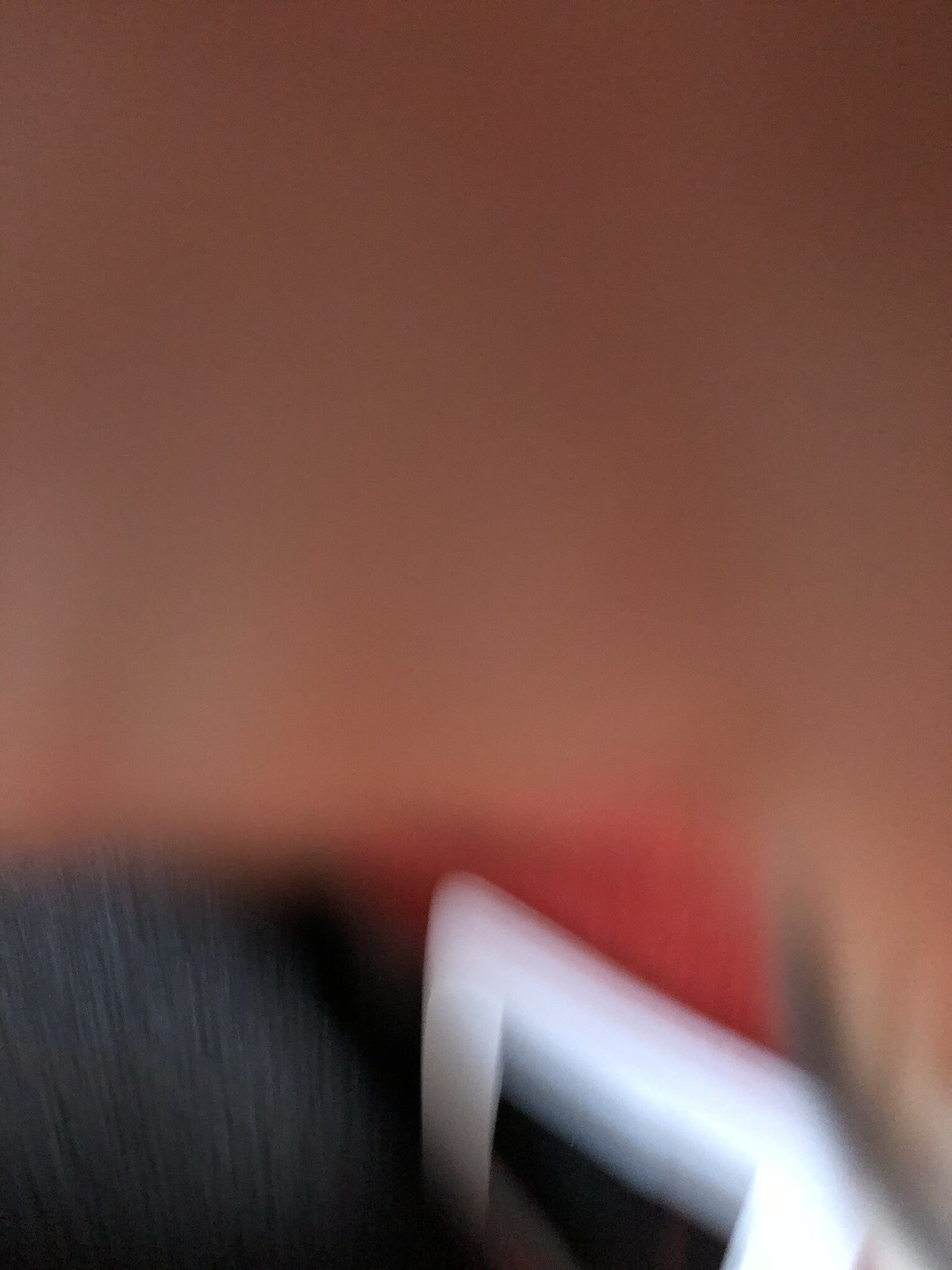The image features a predominantly blurred close-up shot with a complex interplay of colors and lighting. The background is primarily brown, transitioning to black near the bottom. The top section of the image continues the brown hue, while the lower left corner has a dark tone. Directly in the center, a patch of red becomes visible, creating a striking contrast against the surrounding colors. The right side of the image includes some white, possibly created by a source of light that also casts illumination across the scene. This white extends to the bottom right corner, though it’s mixed with other colors and bright spots likely due to the lighting effects. The lighting originates from the right side, casting two distinct, albeit subtle, beams across the scene. Amidst the diffuse colors and blurred forms, a small white segment is discernible at the bottom left, possibly reflecting light. The red patch mentioned earlier is also more pronounced near a corner, adding a focal point amidst the ambiguity. Overall, the visual details remain obscure due to the heavy blur, making it difficult to discern specific details or objects.